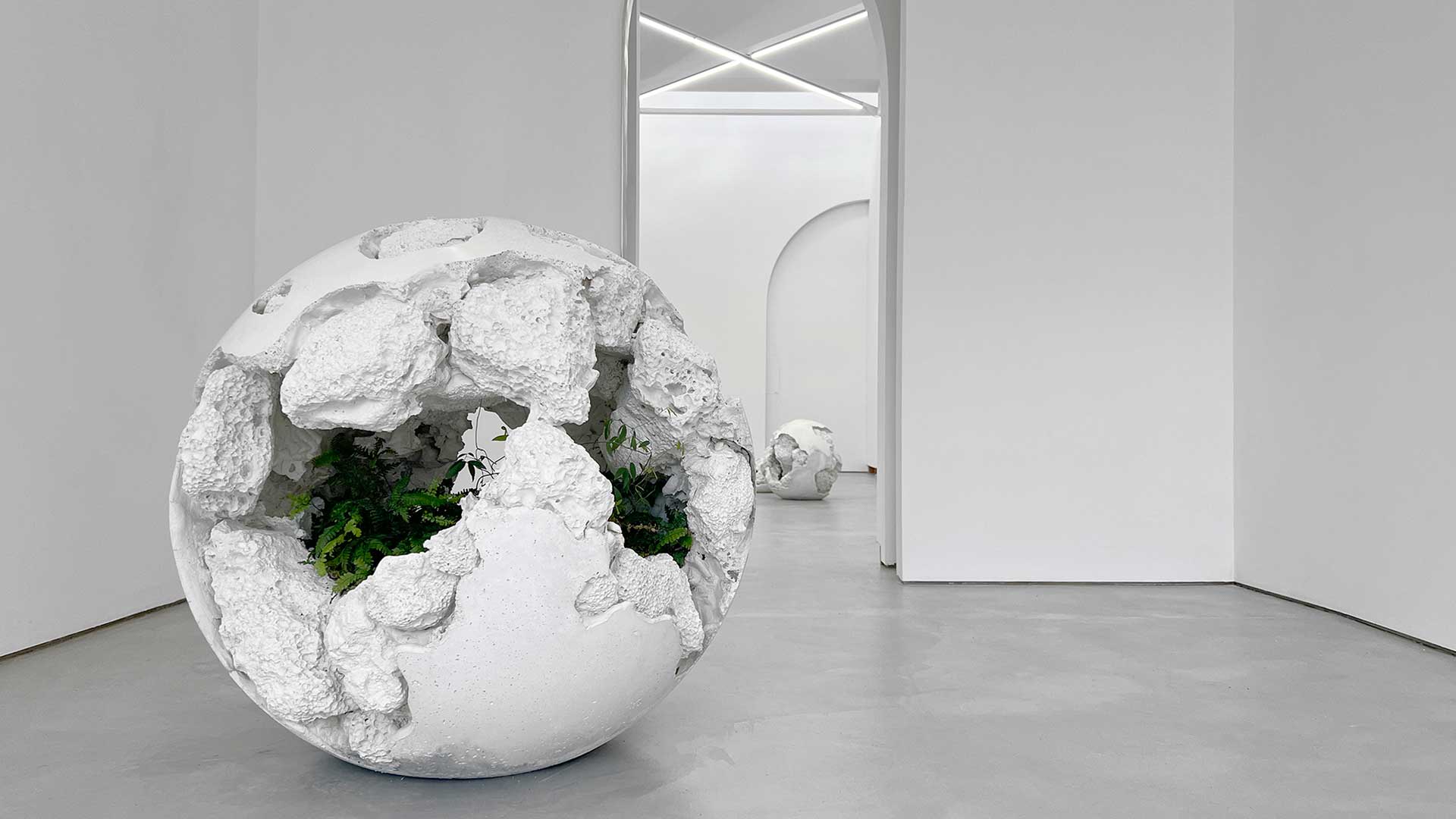The image displays a modern, minimalistic room with solid white walls and a gray floor. The walls are unadorned and devoid of any paint or decorations. The focal point of the room is a cracked, spherical sculpture that catches the eye with its intricate details. The sphere has jagged edges where it is broken, revealing an intriguing interior. Emerging from the cracks are vibrant green plants, with their leaves contrasting sharply against the smooth surface of the sculpture. There is a clear walkway leading to another part of the room, where a second spherical sculpture can be observed. This sculpture is also cracked and jagged, but due to its orientation, the interior details aren't visible.